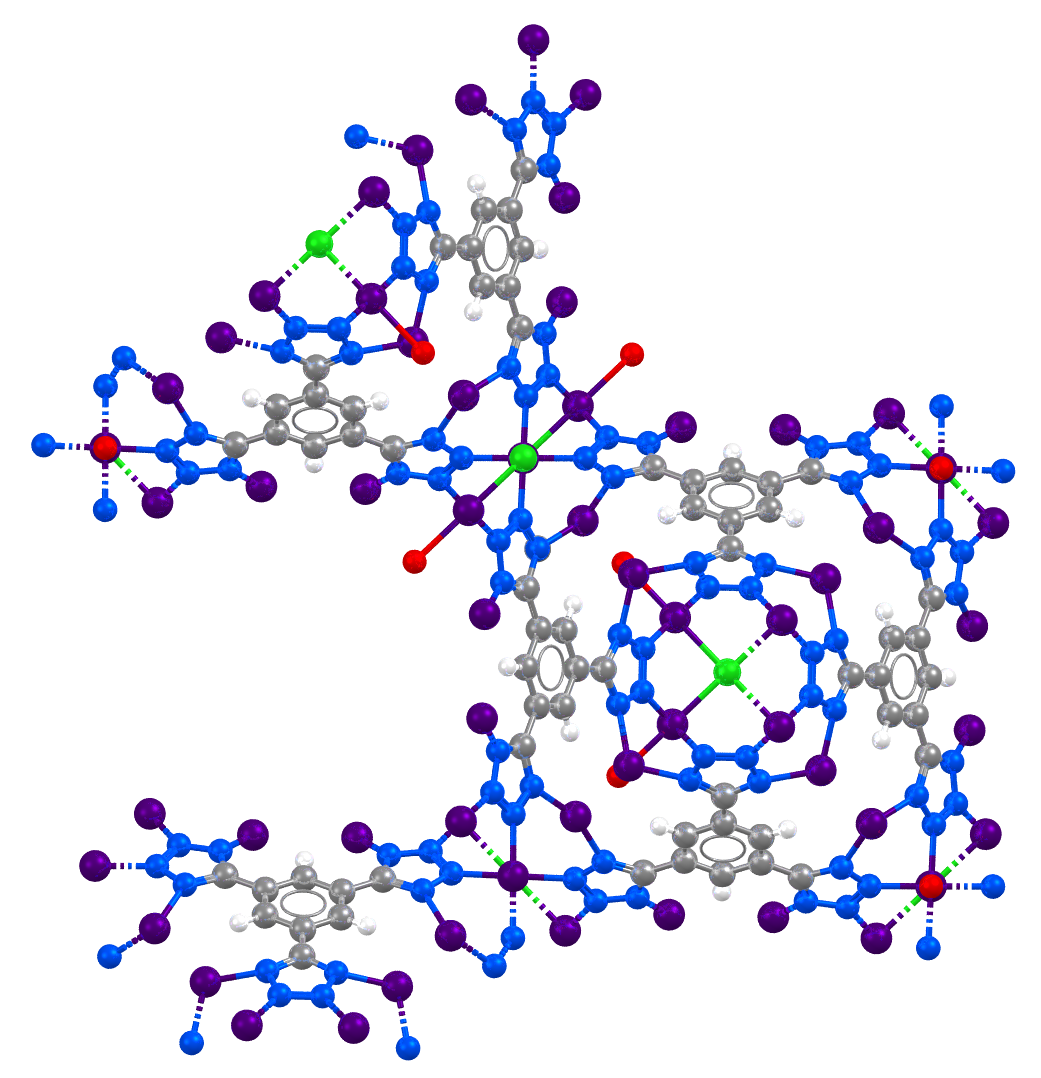The image depicts an abstract representation of a chemical or molecular structure, primarily designed for educational or scientific purposes. It features numerous marble-sized spherical shapes in a variety of colors, including silver, royal blue, light blue, dark blue, purple, lime green, neon green, red, and gray. These spheres are interconnected by lines that vary in color, forming different geometric configurations such as cubes, triangles, and possibly snowflake-like patterns. There are approximately 9 to 10 distinct shapes within the structure, all intricately linked. Set against a clean white background, the image lacks any accompanying text, leaving the viewer to interpret its scientific context or appreciate its artistic quality.